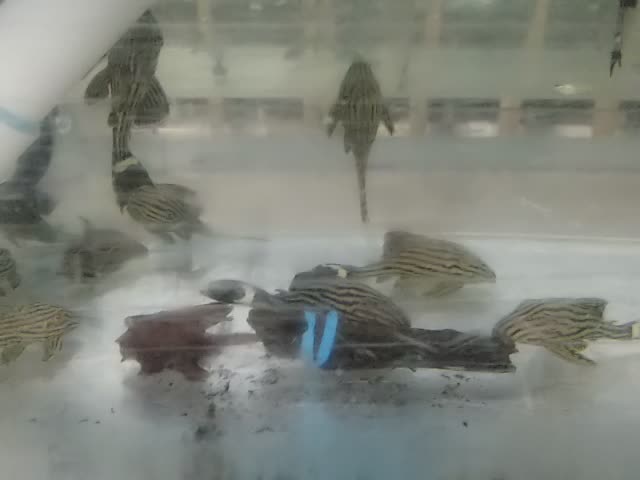This is a slightly blurry color photograph capturing a scientific-type holding tank, likely in a facility that sells fish. Prominently displayed are several Zebra Danios, identifiable by their light brownish beige bodies adorned with distinct horizontal rippling dark brown stripes. These fish are set against an undecorated, muted background within the tank. Among the Danios, a goldfish is also visible, adding contrast to the scene. We can discern additional tanks aligned along a wall in the background, suggesting the setting is a larger setup with multiple aquatic habitats. The tank's interior is sparse, featuring just a few darker objects and possibly a piece of wood with turquoise strips, adding minimal decor to the environment. The photograph's muted colors and slight blur obscure some details, including a light blue U shape, which could be a feature of the tank or an element attached to one of the fish. Overall, the image provides a detailed yet slightly ambiguous view of these tropical fish in a commercial or scientific aquarium setting.